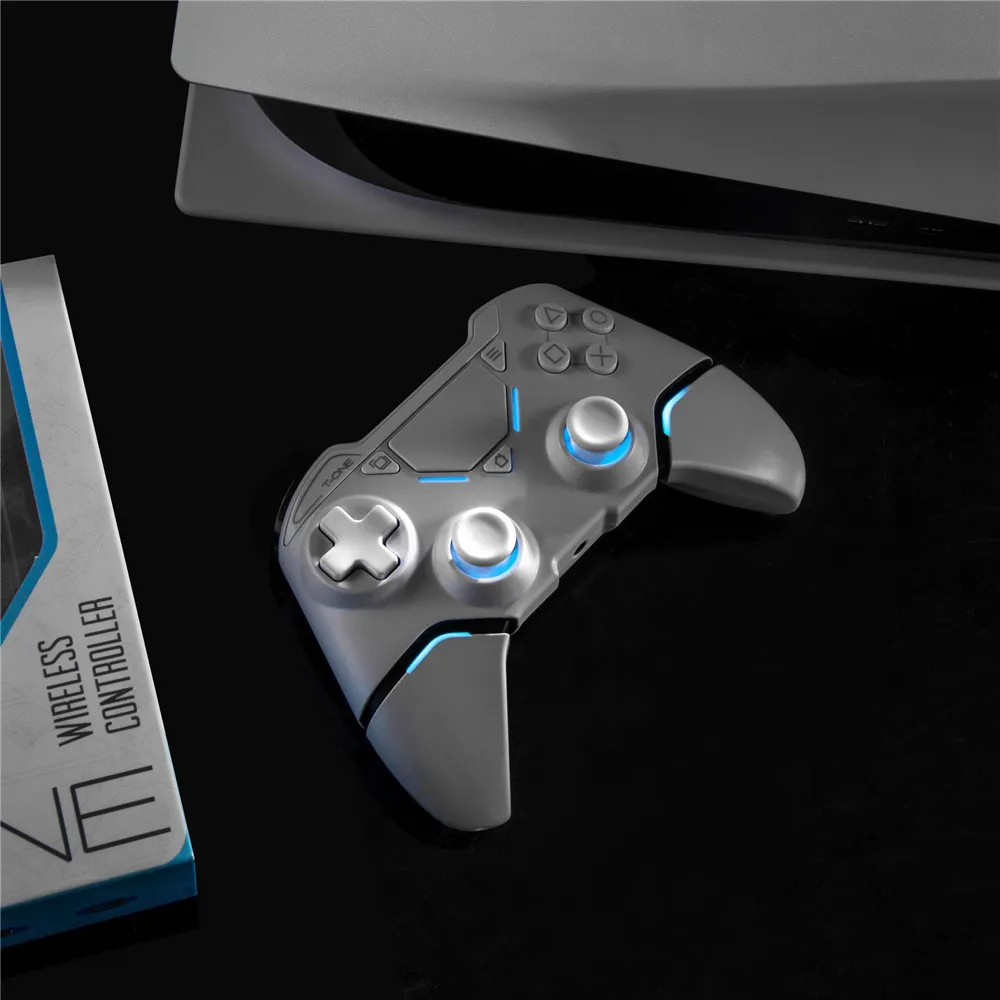This is a detailed image of a gray wireless PlayStation 5 controller set against a plain black background. The square image measures approximately 5 inches by 5 inches. The central focus is the controller, which is long and rectangular at the top with two beveled triangle grips extending downward. These grips are designed to be held by both hands, with joysticks placed at the bottom center for thumb operation.

The controller features bright blue lights emanating from beneath the joysticks and along other sections. On the left side, there is a D-pad, characterized by a plus-shaped design that facilitates directional movement. On the right side, four buttons are arranged in a diamond pattern, labeled with distinctive PlayStation symbols: a triangle, circle, square, and X.

In the lower left portion of the image, partially visible, is a white box with blue outlines and black print that reads "Wireless Controller." Additionally, at the top of the image, part of the PlayStation 5 console can be seen, distinguished by its white exterior and black glossy interior, recognizable by two thin flat layers of gray plastic with an open black area in between.

Overall, this image focuses on the intricate details and design of the PlayStation 5 wireless controller along with a glimpse of the PS5 console, all set against a stark black background.